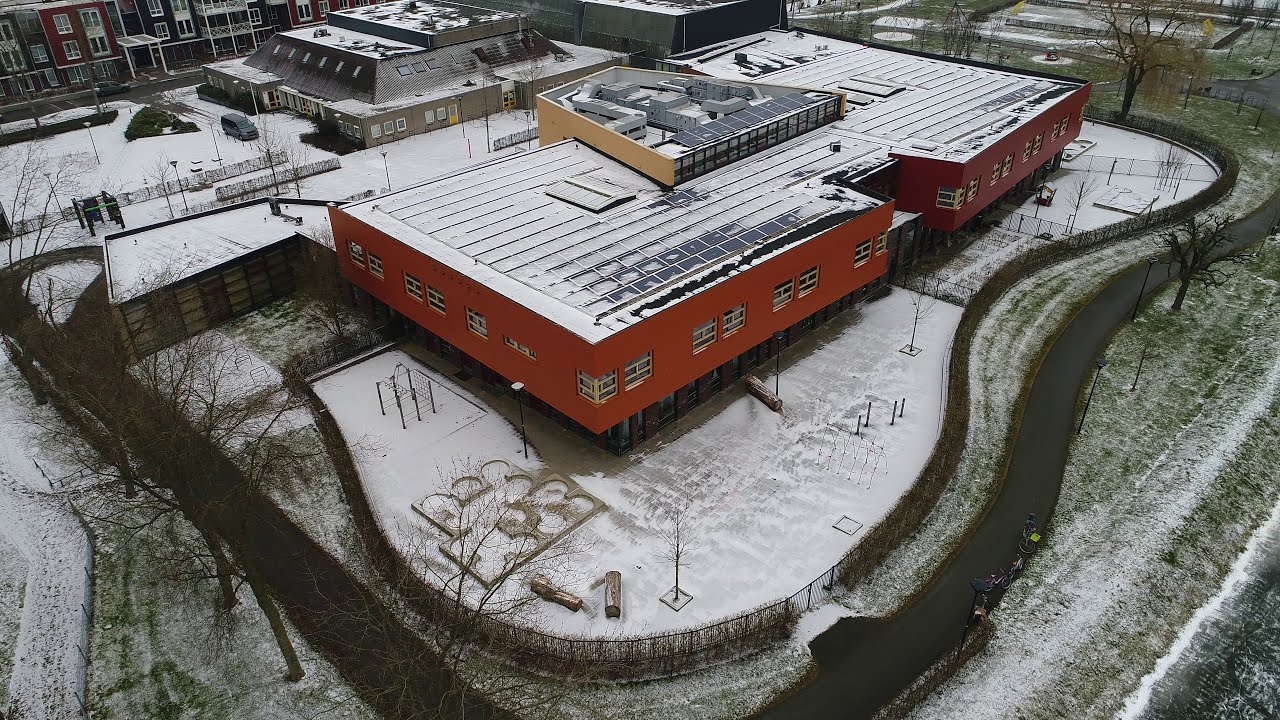The image depicts a striking aerial view of a square, single-story red building, likely a school, situated centrally in a winter landscape. The flat roof of the building is blanketed in white snow, mirroring the snow-covered yards and surrounding areas. Numerous large windows punctuate the sides of the building. Flecks of green grass peek through the snow, hinting at the dormant lawn beneath. Various playground equipment scattered around the yard further suggest the building’s educational purpose. Encircling the building, a dark black asphalt road straightens out toward the bottom left and curves gracefully around the bottom right. In the background, additional gray, pyramid-like structures with flat tops are visible, enhancing the scene's architectural diversity. Trees scattered around the scene add a natural element to the otherwise structured environment, highlighting the harmony between the built and natural worlds even in winter’s embrace.